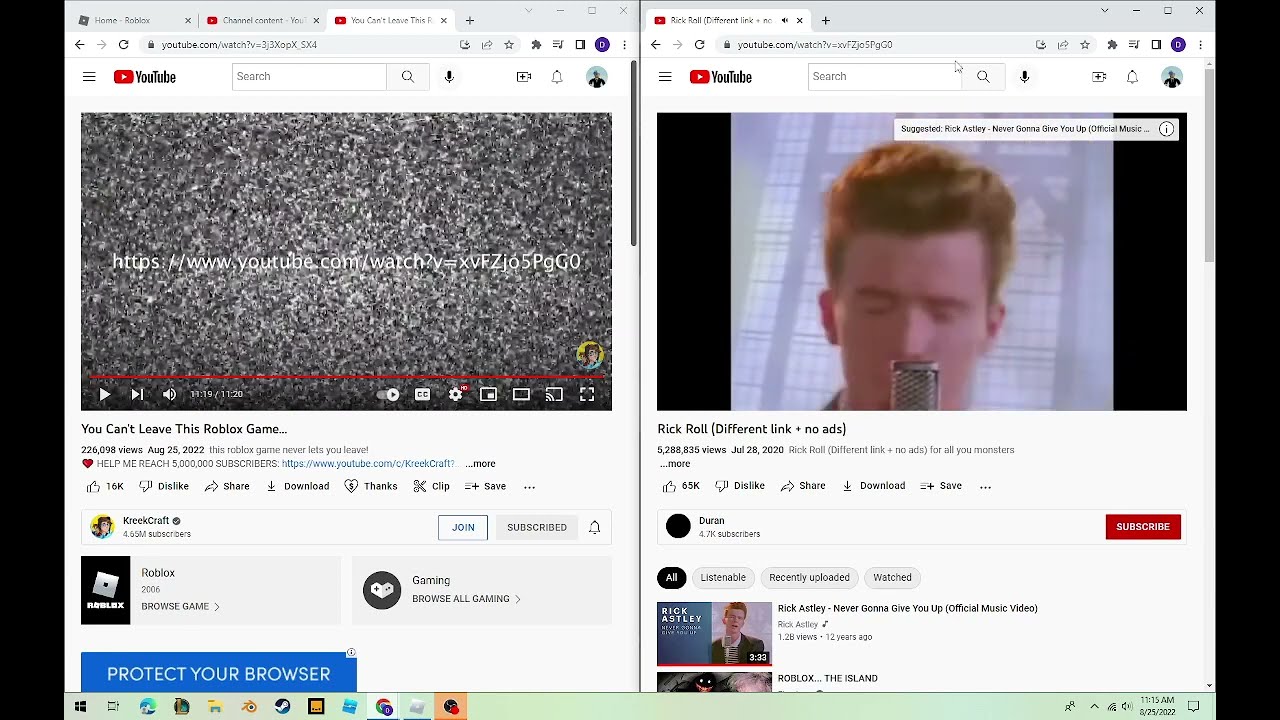The image displays a juxtaposition of two YouTube videos with a humorous twist. On the left, there is a video titled "You Can't Leave This Roblox Game..." which has garnered over 220,000 views since its release in August 2022. The video description includes a URL, enticing viewers to click it. On the right side, the image reveals the destination of that URL—a classic Rickroll video titled "Different Link, No Ads" which has been visited by over 5.2 million people. The entire setup is a playful prank where the first video purports to show a Roblox game that traps players, but in reality, directs them to the Rick Astley music video, a well-known internet meme used to troll viewers. This clever ruse has successfully duped over 200,000 individuals into experiencing the timeless meme.